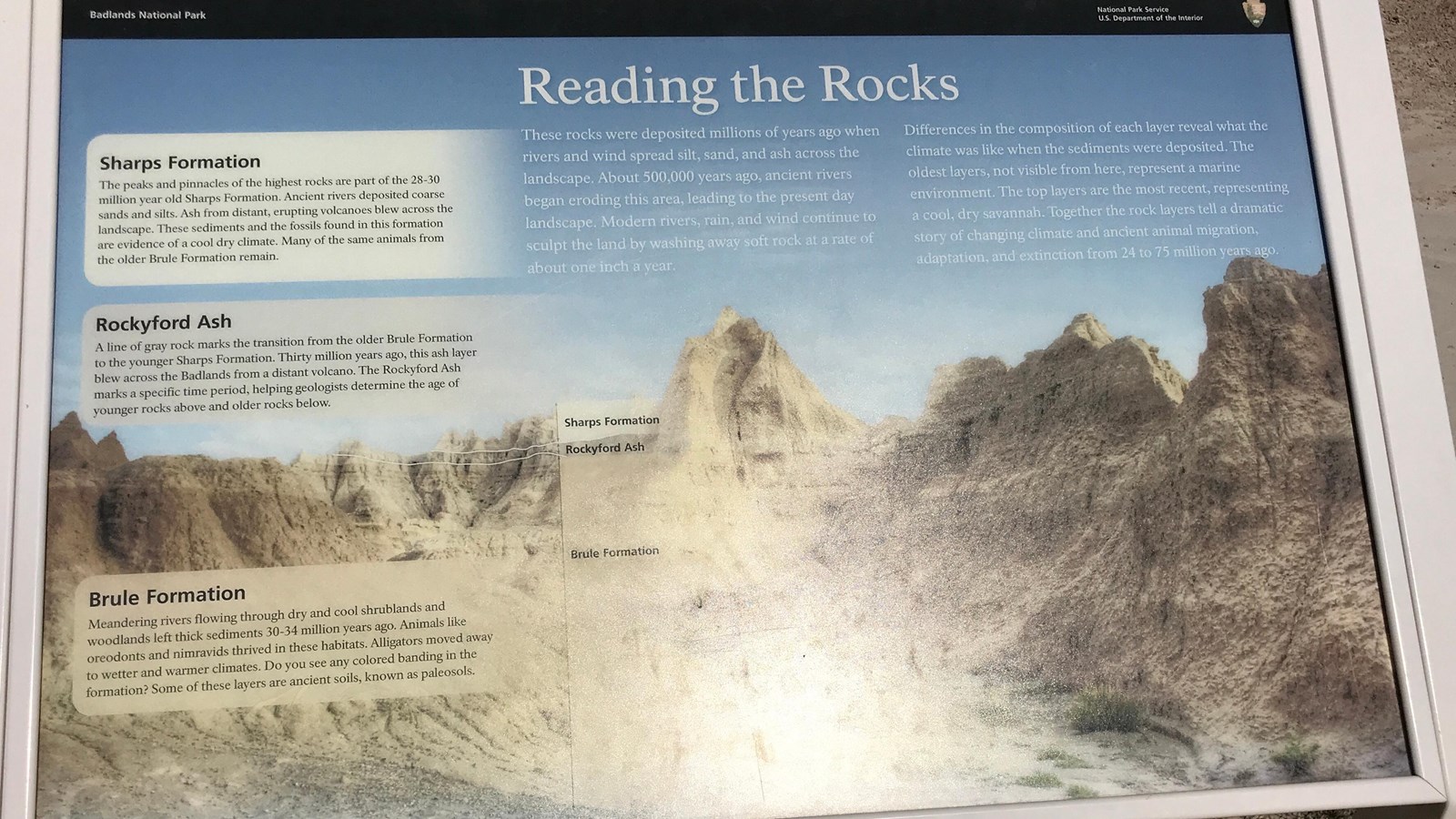The image is an up-close photo of an informational plaque encased in a silver metal border. At the top of the plaque, a thin black horizontal strip displays the name "Badlands National Park" on the left and the logo of the National Park Service, U.S. Department of the Interior, on the right. The central headline reads "Reading the Rocks" in large white letters over a blue sky background with tan, sharply rising hills.

The plaque provides a detailed explanation of the geological history of the Badlands. It states that these rocks were deposited millions of years ago as rivers, wind, and ash spread sediment across the landscape. About 500,000 years ago, ancient rivers began to erode the area, shaping the present landscape, which continues to change as modern rivers, rain, and wind scour the land, eroding soft rock at about one inch per year.

Beneath the headline is a detailed narrative, explaining that the differences in rock layers reveal the climate when sediments were deposited. The oldest layers represent a marine environment, while the topmost are from a cool, dry savannah. The rock layers tell a story of dramatic climate changes and ancient animal migrations from 24 to 75 million years ago.

The plaque includes images and descriptions of three major formations: 
1. **Sharps Formation**: Peaks and pinnacles from 28-30 million years ago, formed by ancient rivers depositing sand and silt, mixed with volcanic ash, indicating a cool, dry climate.
2. **Rockyford Ash**: A gray ash layer from 30 million years ago, marking the transition from Brule to Sharps Formations, helping geologists determine the age of the rock layers.
3. **Brule Formation**: Deposits from rivers in dry, cool shrublands 30-34 million years ago, rich in fossils of animals like oreodonts and nimravids, with alligators moving to wetter climates.

On the left of the plaque, there are additional images of rocks with annotations, further elaborating on the characteristics of these formations, showcasing the varied geological history and the ongoing natural processes shaping the region.